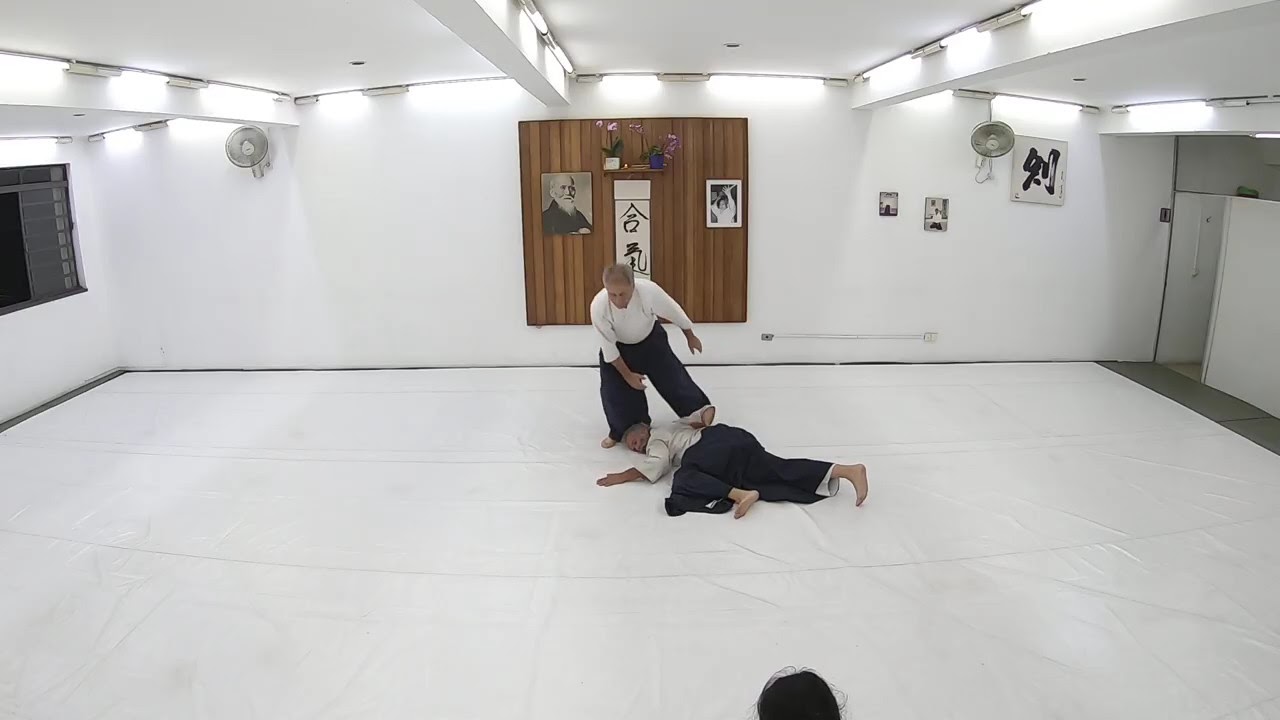This rectangular indoor photograph captures a serene and disciplined dojo, entirely adorned in white, from the padded floor to the walls and ceiling. A wooden plank section on a rear wall hosts a shelf with orchids, Asian calligraphy, and portraits suggestive of martial arts mastery. Centerstage on the pristine white mats are two men engaged in what appears to be martial arts or self-defense training. Both are attired in traditional martial arts uniforms with black pants and white crossover tops. One man, an older individual with gray hair and dark skin, is lying face down with his limbs outstretched, possibly simulating an injured state. The other man bends over him, mid-movement. Observing this scene, a third figure's head is slightly visible at the photo's bottom center. The calm and disciplined atmosphere is accentuated by additional elements like hanging fans, lighting, and a single window, creating a striking and authentic representation of a martial arts environment.